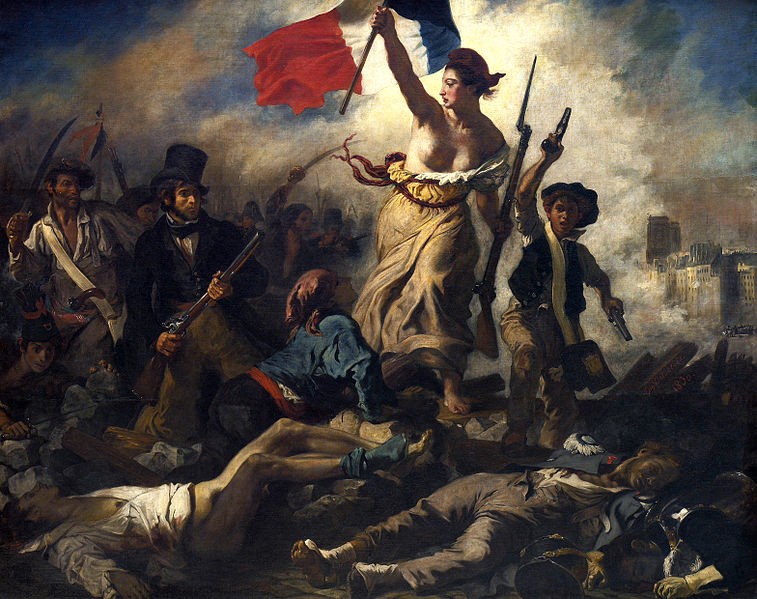The painting depicts a dramatic and intense scene from the French Revolution. At the center is a woman in a beige, goldish dress with part of her breasts exposed. She holds the French tricolor flag, red, white, and blue striped, high in her left hand, symbolizing freedom and revolution. Around her, the ground is littered with bodies in blue overcoats, brownish pants, and white tops, indicating the fallen soldiers. To her right, a young man wields two pistols, and nearby, a figure in a black top hat brandishes a shotgun. Behind them, another man with a sword dons a light blue shirt. The backdrop features indistinct figures and billowing smoke, creating a chaotic atmosphere. The woman is prominently highlighted against a whitish cloud of smoke, emphasizing her leadership and the tumultuous victory.